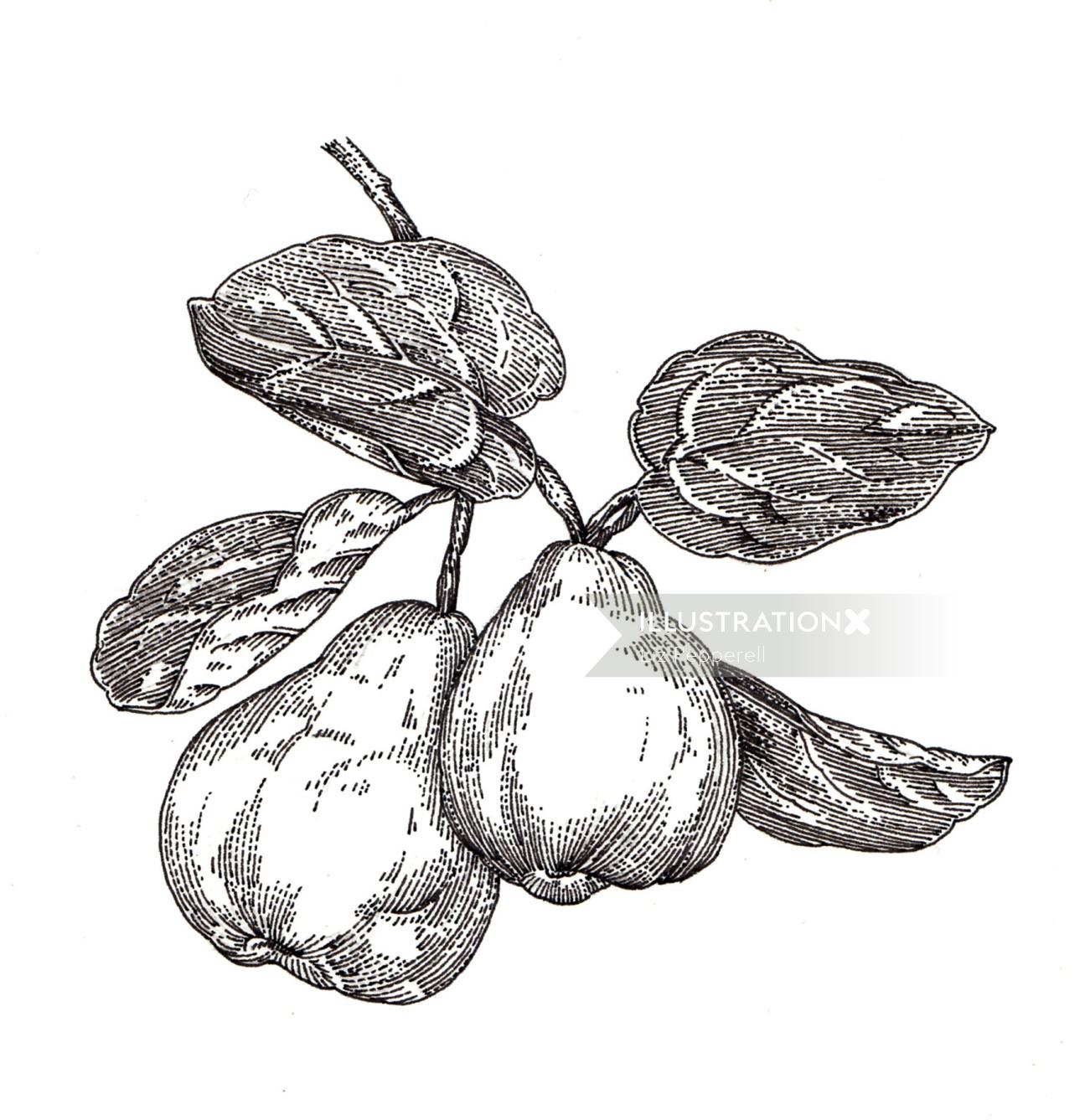This image is a detailed, black and white drawing of two pears created by the program called Illustration X. The pears, one larger than the other, are shown still attached to branches with several jagged-edged leaves surrounding them. The image is entirely in grayscale, showcasing variations in shading through pencil or charcoal techniques, making it appear hand-drawn. A gray banner cuts across the middle of the drawing, displaying the text "Illustration X" in white lettering. The leaves are filled with dark shading, providing contrast against the white background. There are no labels or context provided to suggest the colors of the pears, leaving their potential hues—whether brown, green, or yellow—up to the viewer's imagination. The drawing is proportionally accurate and meticulously detailed, particularly in the leaf variegation and the natural curvature of the pears.